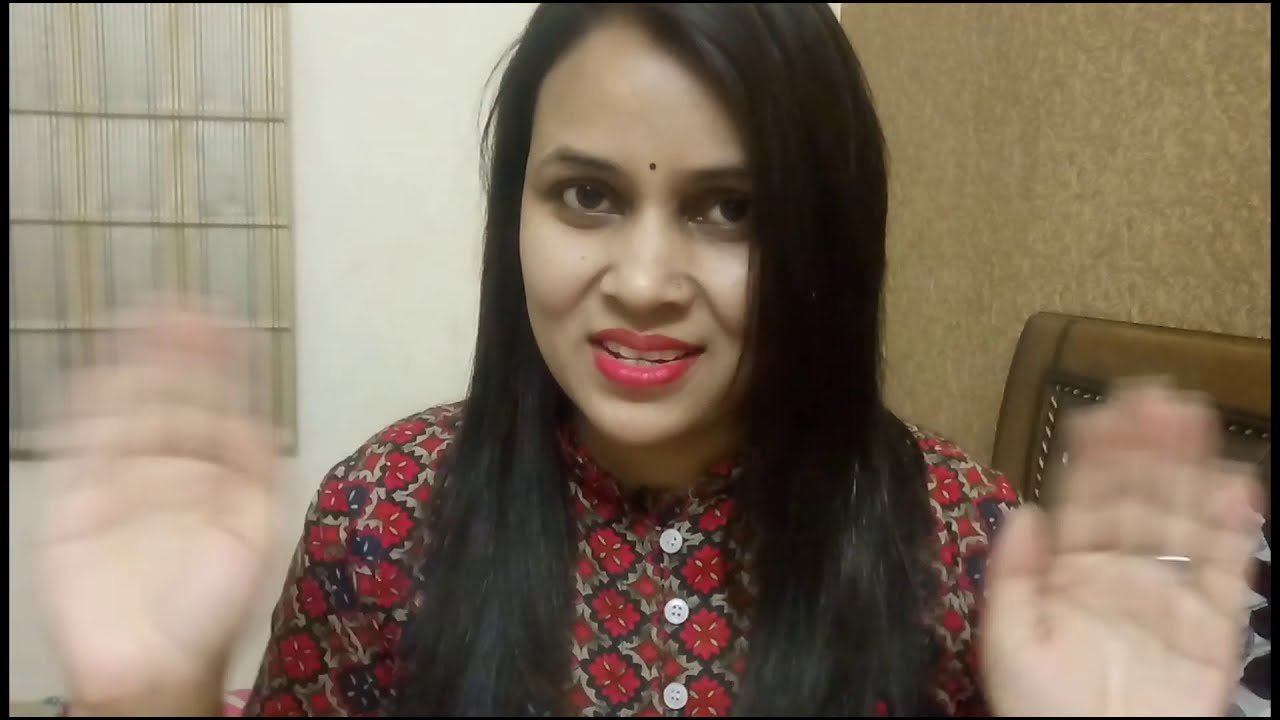The photograph depicts a young Indian woman with long, straight dark brown hair that frames her face by swooping over to the left side. She has a light brown complexion, prominent cheekbones, and dark eyes. She is wearing deep magenta lipstick and has a bindi on her forehead. She is engaged in a video call, possibly via Skype or FaceTime, and is captured from the chest up. Her mouth is open, revealing part of her upper and lower teeth, suggesting she is in the middle of speaking. She wears a high-necked, button-up shirt with a red and black paisley-like repeating pattern, featuring three pearl buttons in the front. Both of her hands are raised with palms facing towards the viewer, appearing blurred as if she is waving them side to side, perhaps signaling to get attention or express a gesture. A gold band adorns her left ring finger. In the background, there is a beige wall with some gray pinstriped artwork and a hotel bed on the right side. The image is a color photograph in landscape orientation.